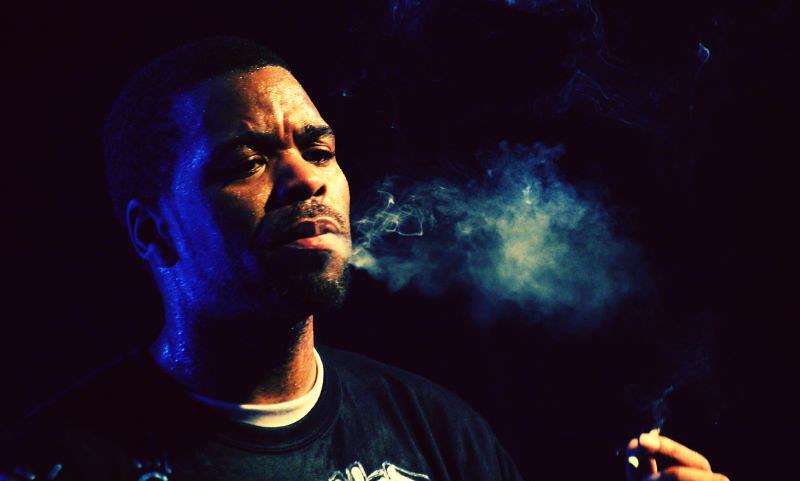In this striking image, a Black man is captured smoking in a dimly lit environment. The left side of the photograph is bathed in a soft blue light, creating a moody contrast against the dark background, while a more direct, clear light illuminates the right side. The man, dressed in a navy blue shirt layered over a white vest, is holding up a cigarette. Wisps of smoke, exhaled from his mouth, trail upwards toward the top right corner of the frame. His face glistens with sweat, and a well-groomed beard frames his contemplative expression as he gazes toward the right side of the image. The interplay of light and shadow, along with the drifting smoke, adds to the atmospheric intensity of the scene.